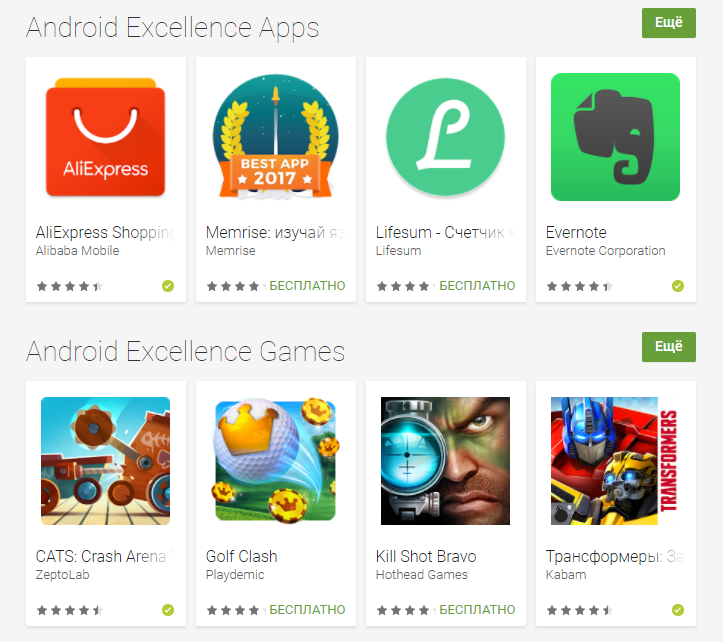This image showcases a page highlighting various Android Excellence apps and games. Prominently featured apps include "Le Express," "Memorize," and "Meme Rise." Additionally, there’s an app with a script that is unrecognizable and labeled as the best app of 2017. Further down, there's "LifeSum," with text that looks similar to Greek or Turkish writing.

Among the highlighted apps, "Evernote" stands out with its amusing logo – a green square featuring the head of a black elephant. On the gaming side, there's "Cats: Crash Arena," noted under the Android Excellence games category. Also mentioned are "Golf Clash" and "Kill Shot Bravo," the latter having a logo with a very unpleasant, glaring face. Another game title is displayed in a script that might be Russian, followed by "Transformers."